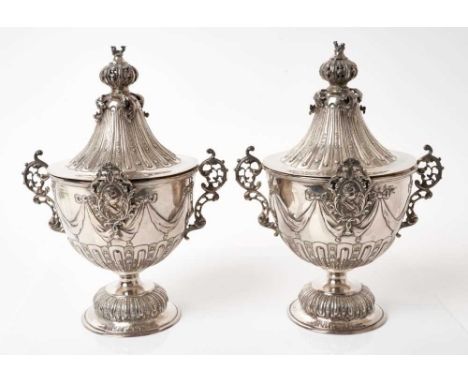This photograph features two stylized, symmetrical urn-like chalices that appear to be antiques or elaborate, expensive pieces. The urns are situated against a plain white background and rest on a white tabletop, split down the center with one urn on either side. Both urns are predominantly silver, with darker silver handles and ornamentation, including small dome-like shapes at the tops of their lids. These lids are pyramid-shaped and bear a striking resemblance to witch's hats, with a round oriental or pumpkin-like ornament crowning each. The urns, which can also be described as goblets, feature intricate filigree designs resembling grapevines and ribbon-like decorations circling around them. The base of each urn is goblet-shaped, complete with a slender stem leading down to a rounded foot, and adorned with striped, linear designs. Both urns are masterpieces of dual-toned silver artistry, blending lighter and darker silvers seamlessly to create a cohesive, ornate appearance.